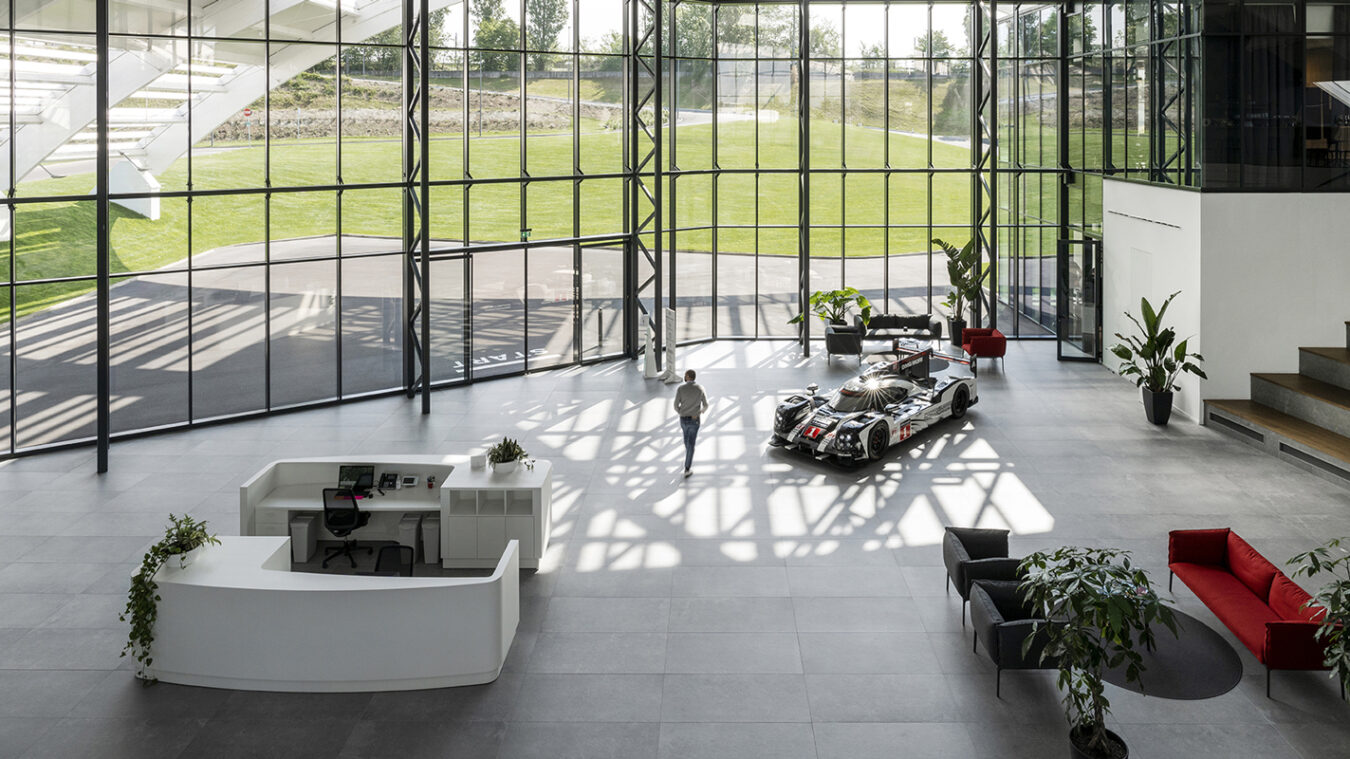The image showcases a modern, spacious office building lobby characterized by its transparent glass walls and high ceilings. The interior is visually striking with its gray tiled floor and numerous plants throughout. Dominating the foreground is a sleek white sports car with black and subtle red accents, featuring red numbers that add a touch of vibrancy. This car appears to be in a showroom-like area. To the right of the car, a waiting area is furnished with a distinctive red couch and two gray chairs, creating a focal point with their bold color contrast. In front of one glass wall, black structural supports divide the glass panes, and beyond it, a lush green lawn and a white external structure are visible. 

A white receptionist desk with a cascading green plant and a black chair is centrally located, complementing the scattered arrangement of several large plants. In the background, the photo hints at an upper level accessible via a set of stairs, with a notable large white structure positioned towards the upper right corner, further enhancing the open, airy ambiance of the lobby.